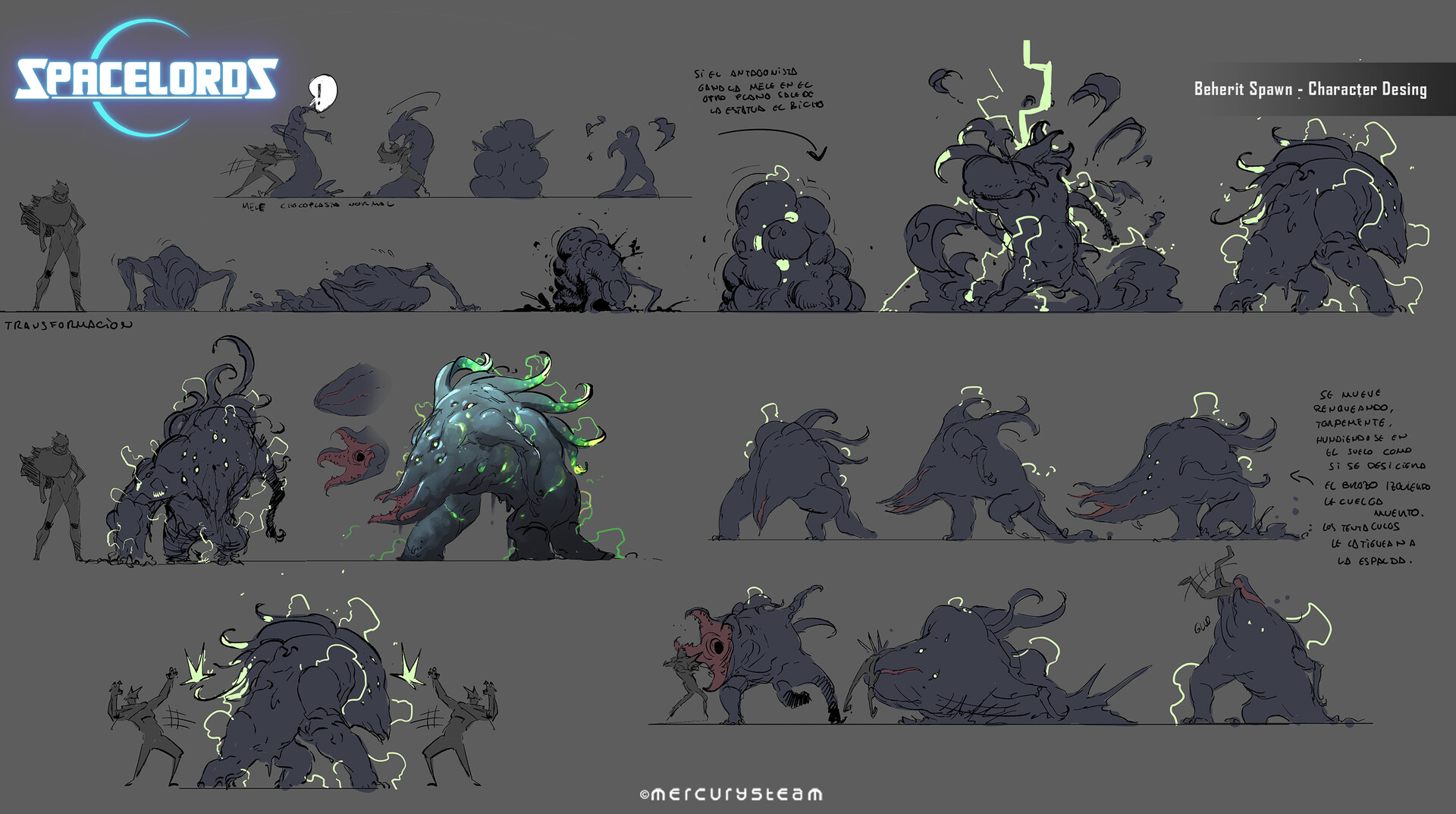The poster, set against a dark gray background, features the title "Space Lords" in the top left corner, with the white font having a subtle purple-blue iridescent hue. The layout is divided into several rows, depicting an evolving storyline through different illustrations. These rows showcase a transformation, where the monster morphs, growing into a more defined character as you move from left to right. The monster, somewhat dinosaur-like with a medical or mechanical twist, has greenish tentacles and is gray in color. Opposing this beast are human-like figures clad in armor, engaged in battle. The creatures and characters appear to be walking or sitting on an underlined surface that suggests land. The poster includes a logo resembling a moon or an eclipse with a bluish tint. Additionally, it has the word "MERCURY STEAM" in the bottom center in white font and more white text in the top right corner. Tiny arrows and accompanying text scattered between the characters enhance the dynamic storytelling of this gaming design artwork.